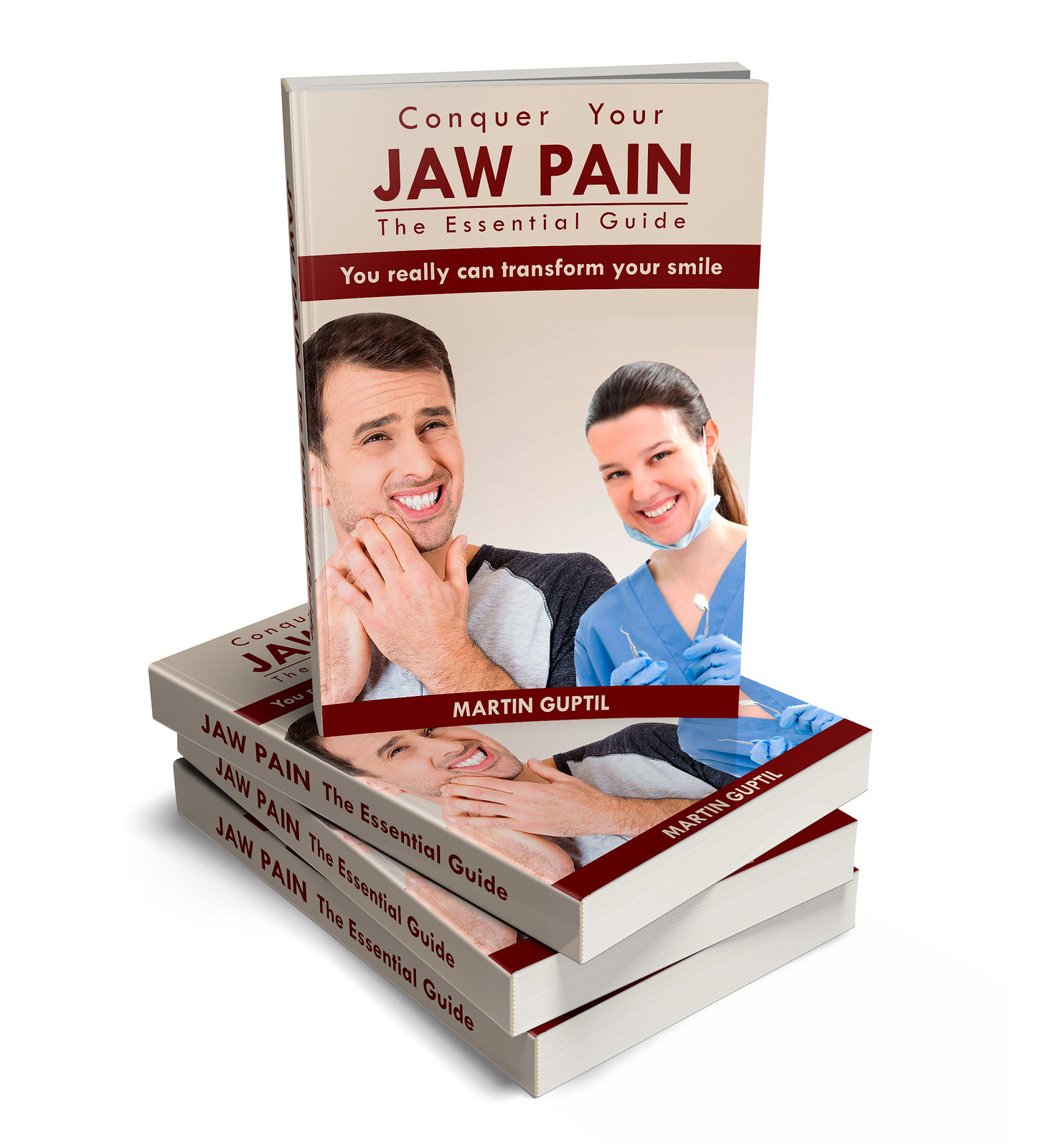This photograph features a stack of four books against a pure white background with a slight shadow at the bottom. Three identical books lie horizontally at the base, their spines towards the bottom left and somewhat askew. On top of these, a fourth copy of the same book is positioned upright, fully visible. The cover of the book reads, "Conquer Your Jaw Pain: The Essential Guide," with a red banner stating, "You really can transform your smile." The author, Martin Guptill, is credited at the bottom. The cover also displays a dual image: a white man on the left holding his jaw in apparent pain and wincing, and a smiling white woman on the right, dressed as a dental professional in blue scrubs with a mask pulled down under her chin, holding dental tools.